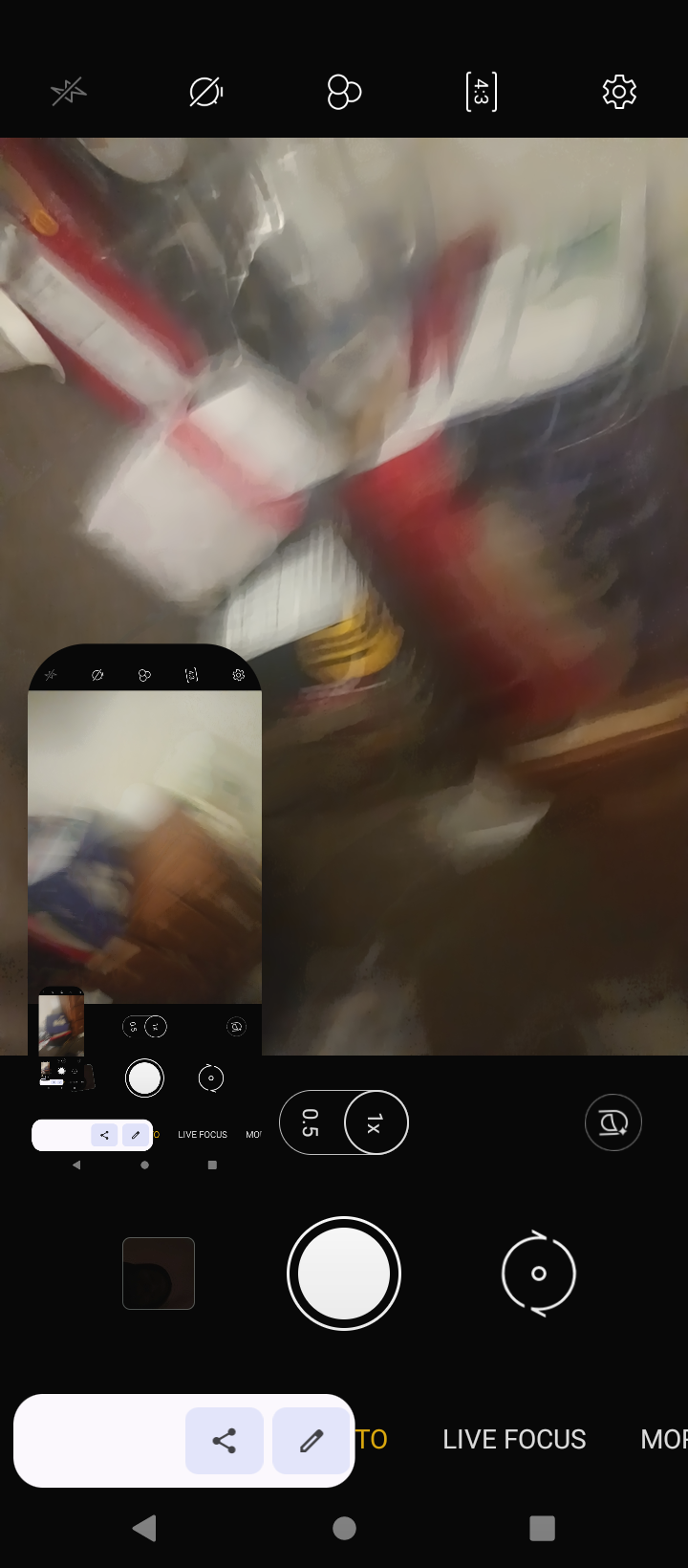This image depicts the interface of a cell phone while taking a video, showcasing a somewhat perplexing and chaotic scene. The main screen displays the typical icons and controls of a smartphone camera, likely an iPhone or a similar device, with the prominent white circle button for recording video at the bottom. To its left, there is a button for switching between front and rear cameras. Visible at the bottom of the screen are various video modes, with "live focus" being the only one clearly legible. There are also some editing tools located on the bottom left of the display.

The primary image on the phone screen is extremely blurry, suggesting the camera might be wet or out of focus, making it difficult to discern specific details. It appears to capture a stack of indistinct, multicolored objects—possibly containers or coolers in red, blue, orange, and yellow—seemingly placed on a countertop or palette.

Inset in the lower left corner of the main image is a picture-in-picture view, showing an even blurrier rendition of the same scene. This smaller image mirrors the primary view with additional distortion, making it resemble a brown package next to a blue one. Above the editing tools at the bottom are typical smartphone navigation icons - a left arrow, a circle, and a square in light gray, as well as sharing and editing options.

Overall, this confusing image combines the standard features of a smartphone camera interface with a highly unclear and indistinct photograph, making it challenging to identify the exact subjects being captured.